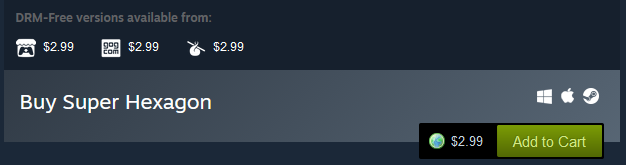This image is a high-resolution screen capture showcasing a digital storefront interface offering DRM-free versions of software or content. At the top, in light gray text, the phrase "DRM-free versions available from" is prominently displayed, followed by a series of icons each labeled with pricing information in off-white text.

- The first icon resembles a small storefront with an awning and a person inside, priced at $2.99.
- The second icon is somewhat unclear, with gray letters and a price listed at $2.99.
- The third icon appears to be a heart symbol with a stick, also priced at $2.99.

Following these icons, a gray box with white font reads, "Buy Super Hexagon," with each word capitalized. To the side, there are icons representing different operating systems: a Windows icon, an Apple icon, and a circular icon possibly indicating another platform or service.

Below these icons, a black box displays a green and blue globe icon with a price of $2.99 and an "Add to Cart" button in green and white. The overall quality of the image is excellent, though the second icon with gray text is slightly difficult to discern. No other noteworthy details are present.